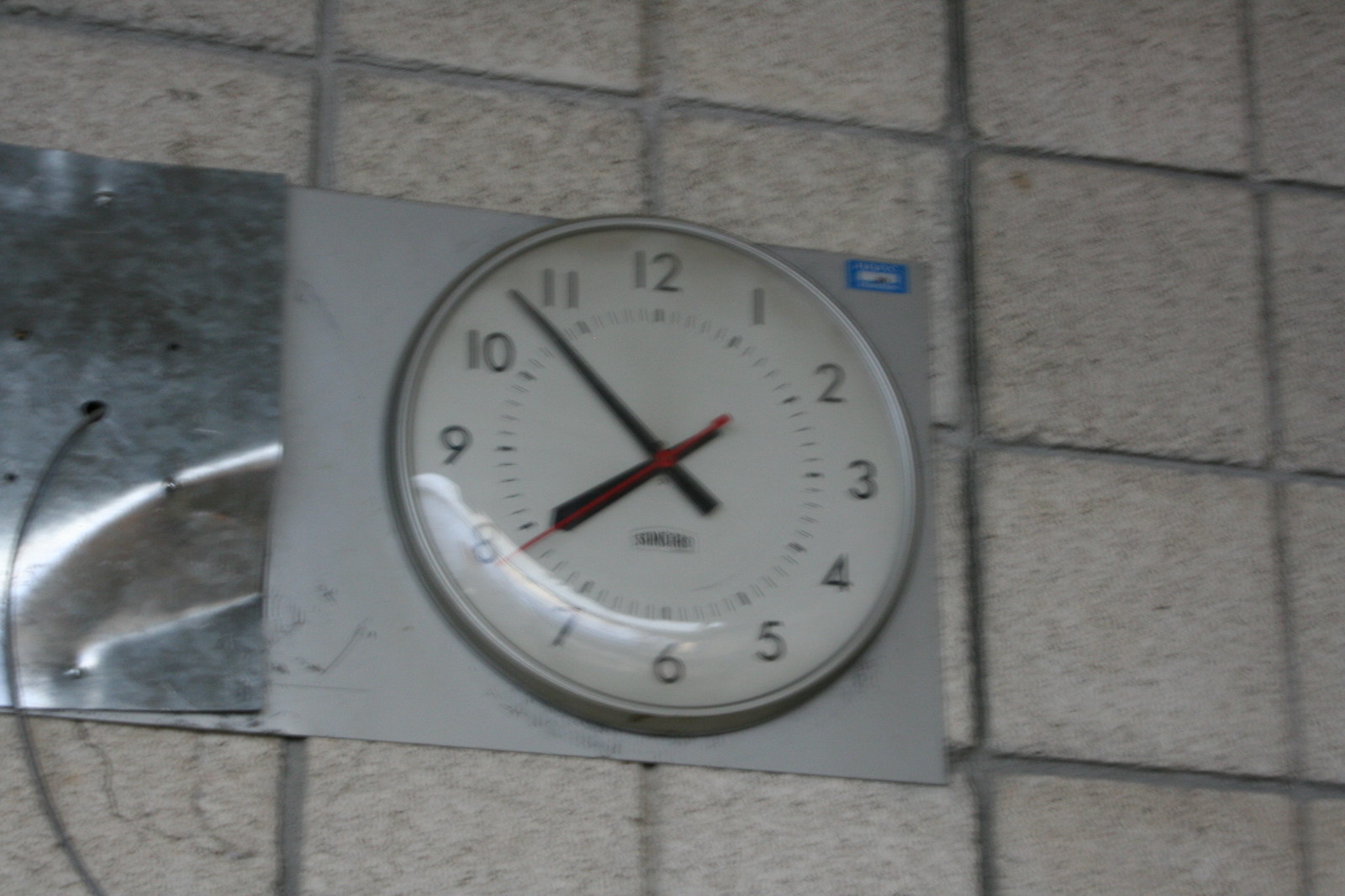This is a photograph of a circular analog wall clock mounted on a silver rectangular plate that is attached to a wall adorned with cream-colored stone tiles. The clock face is white with black numbers, and there is an inner ring of minute markers positioned between the numbers and the center, rather than on the outer rim. The clock features a silver-gray frame, black hour and minute hands, and a red second hand. The wall tiles are a cream marble with specks of black and dark gray, separated by dirty-looking dark gray grout. To the left of the clock, there's a bright silver plate with a wire coming out of it. The clock appears somewhat blurry in the photograph, making the name on the face under the center difficult to discern, though it seems to say "standard." The minute hand is just before the eight, the hour hand is just before the eight, and the second hand is just before the eleven.